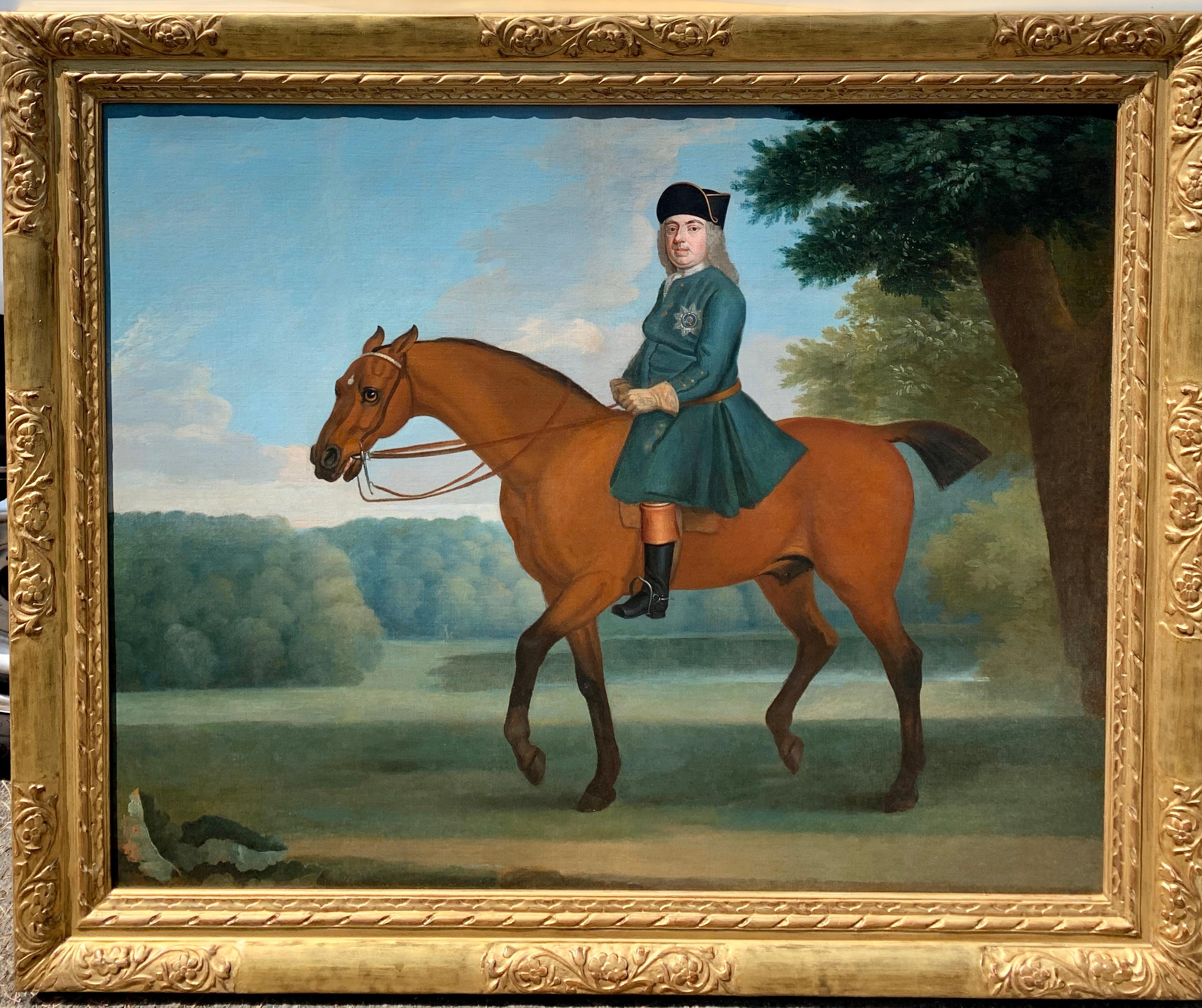This is a detailed painting, framed in an ornate, gilded gold frame with intricate floral etchings at the corners and midpoints. The portrait captures a mid-18th-century scene featuring a person on a horse, likely from the Renaissance or medieval period. The rider, positioned centrally, is dressed in a long blue coat, black riding gloves, and black boots accented with tan at the top. A black hat adorns their head, and long, shoulder-length white or gray hair flows beneath it.

The horse is light brown with a black mane and a notably short-cut tail. It appears to be trotting, with its lead front leg and back right leg in mid-air while the other two legs remain on the ground, suggesting a dynamic motion. The horse's head is turned to the left with a somewhat worried expression. 

The background features a natural landscape with green trees and bushes, providing a serene contrast to the active foreground. A tree on the right side of the painting extends its dark green leaves upward, while a tree line stretches across the image's lower background. hints of water add depth to the scene, and the sky above is a mix of blue with scattered white and gray clouds, enhancing the timeless, pastoral setting.